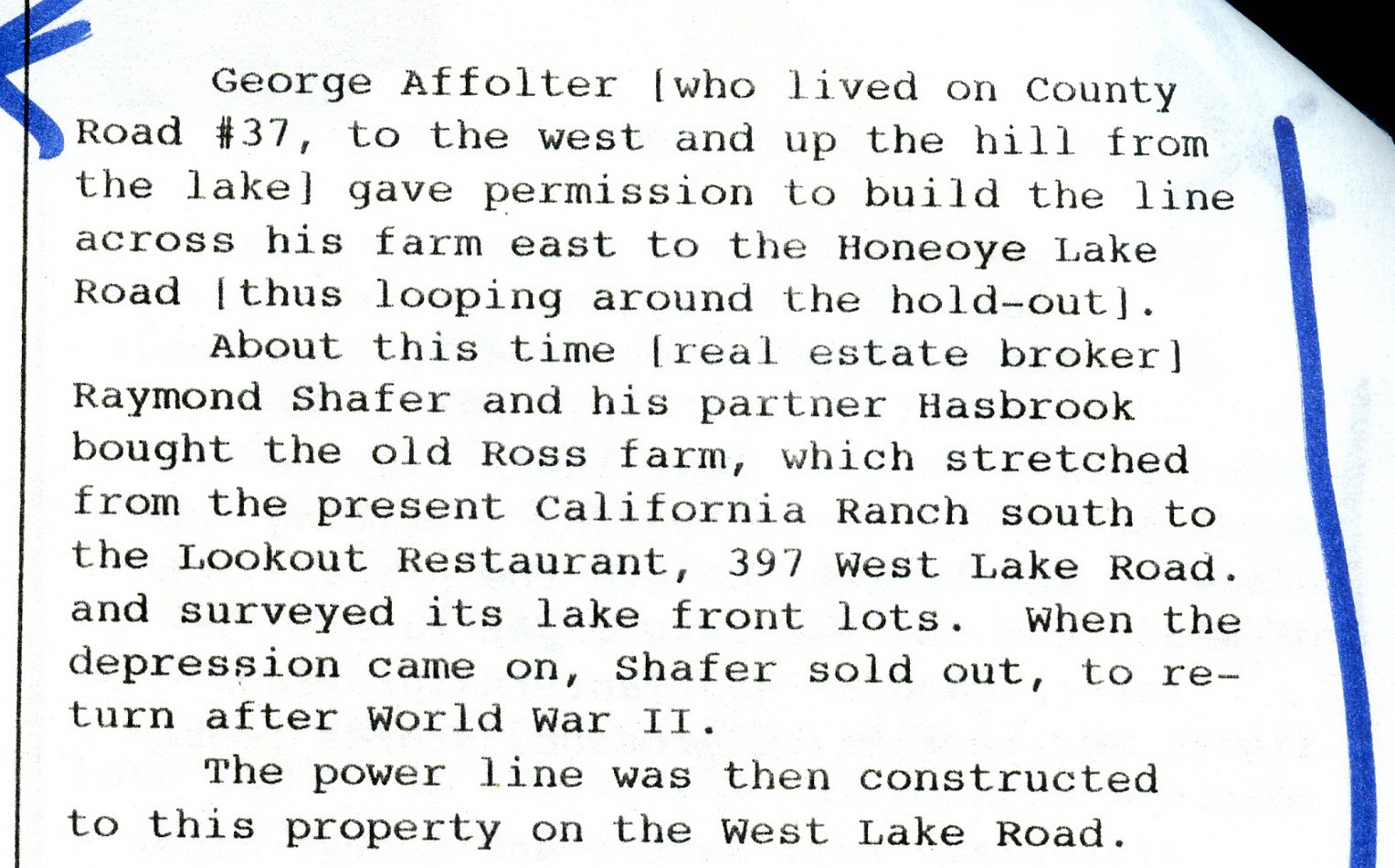The image depicts a typewritten paragraph against a white background, focusing on a historical account involving land transactions and property developments. The paragraph starts with "George F. Falter, who lived on County Road number 37 to the west and up the hill from the lake, gave permission to build the line across his farm east to the Honey Lake Road, thus flipping around the holdout." It continues to describe how real estate broker Raymond Schaefer and his partner Hasbro acquired the old Ross farm, which extended from the present California Ranch south to the Lookout Restaurant at 397 West Lake Road. They surveyed its lakefront lots, but during the Depression, Schaefer sold out, only to return after World War II when the power line was constructed to this property on the West Lake Road. The right side of the article is marked by a vertical blue line, and a small caret on the left suggests to read this passage.